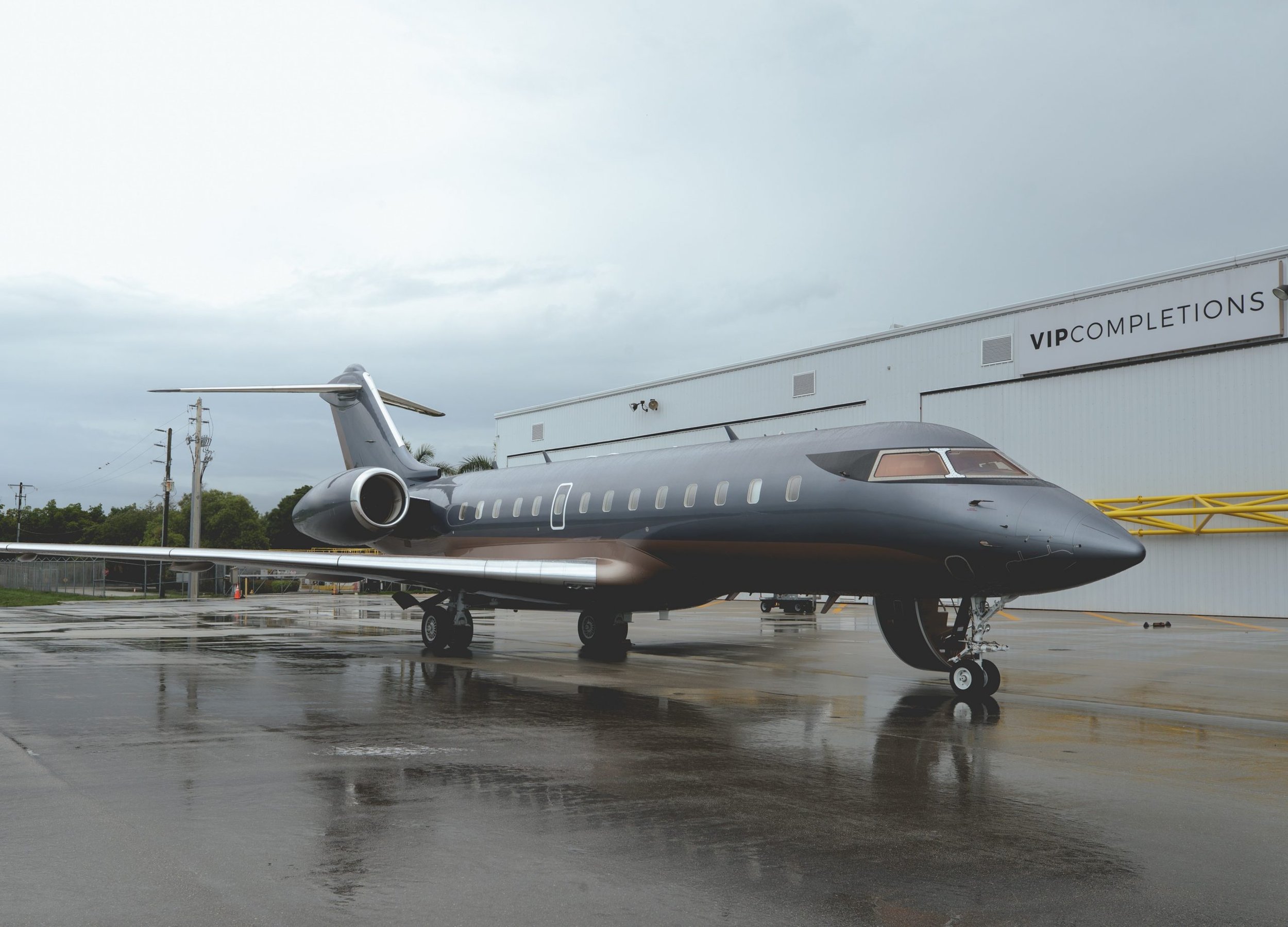The photograph captures a sleek, gray private jet on an overcast day, prominently centered on a wet runway. The airplane's polished concrete-colored exterior, with a hint of silver-blue steel, stands out against the backdrop of gray skies. The aircraft, slightly angled to the right, displays its right wing and rear tail fins, extending out of the frame. Several windows line the side of the jet, accompanied by a white door near the wing. The landing gear is deployed, with two sets of wheels at the back and one at the front under the nose. Surrounding the runway, puddles reflect the recent rainfall, further emphasized by tall light posts and distant trees. On the right side of the image, a large white building, marked "VIP Completions" in black letters, stretches beyond the plane. This hangar, with its closed gates, is accompanied by power lines and a yellow steel structure, completing the industrial setting.